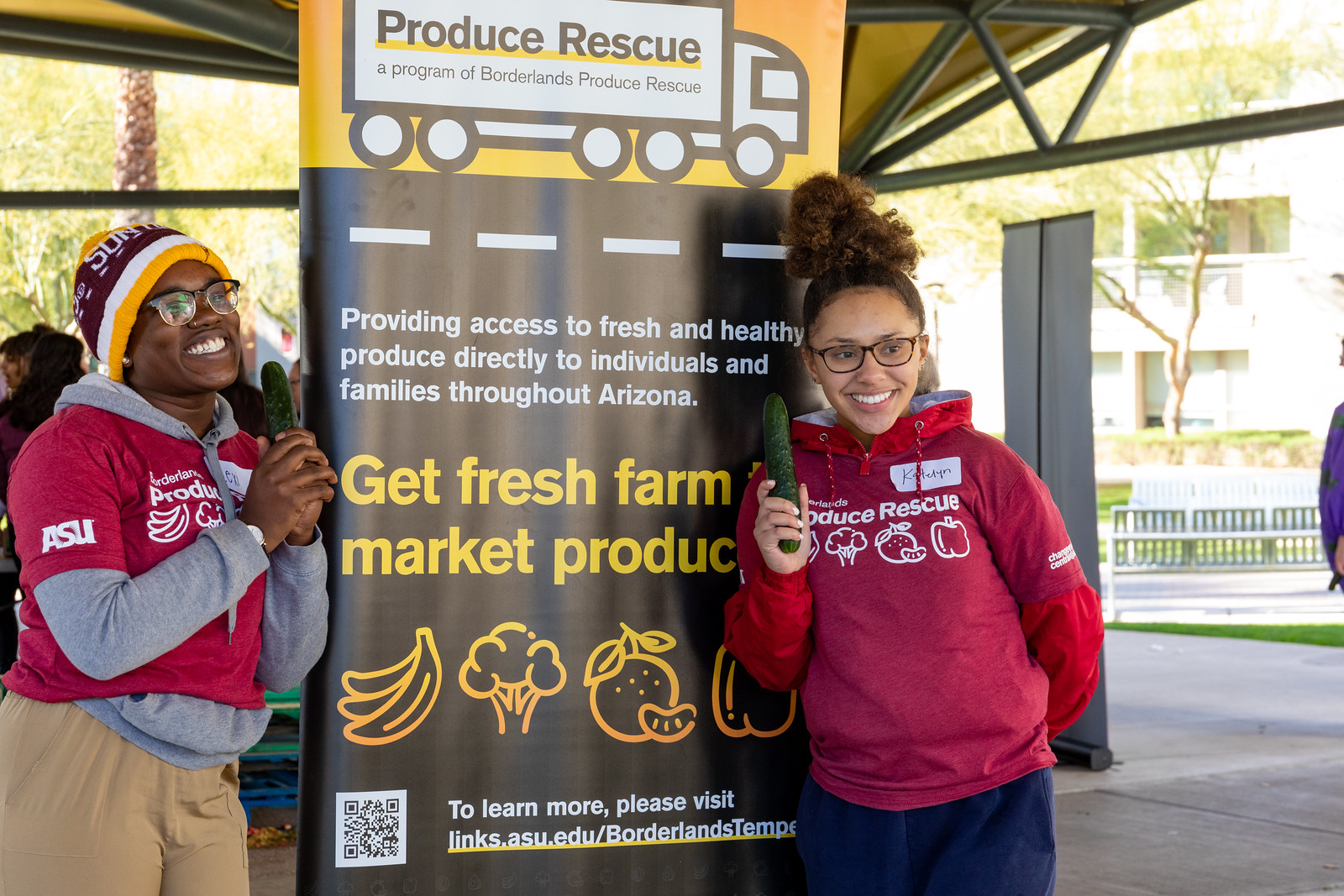In this horizontally aligned rectangular photograph, two young African American individuals are standing in front of a colorful banner on a wall under a covered pavilion. Both are wearing glasses and red shirts branded with the "Produce Rescue" logo, which also displays ASU in yellow and features outlines of various fruits and vegetables such as peppers, oranges, broccoli, bananas, and apples in white ink. The individuals are holding cucumbers up as if they are microphones and smiling towards the right, exuding a playful and cheerful spirit.

The detailed banner indicates that this is part of the Produce Rescue program, an initiative by Borderlands Produce Rescue. The logo of the program is prominently displayed on the image of a truck, and there are white dashes on a brown background below it, mimicking a road. Beneath this, a white text block reads “providing access to fresh and healthy produce directly to individuals and families throughout Arizona.” Below that, in large yellow letters, it says "Get Fresh Farm," though the rest is partially obscured by one of the volunteers, indicating it likely mentions a market or produce-related term. The lower section of the banner also features a QR code and an informative note in white text inviting viewers to learn more by visiting links.asu.edu/borderlandsTempe.

The setting appears to be an outdoor area with a gold-colored tarp for the roof, supported by black bars. In the background, some buildings, benches, a walking path, and touches of greenery are visible, contributing to the lively atmosphere.